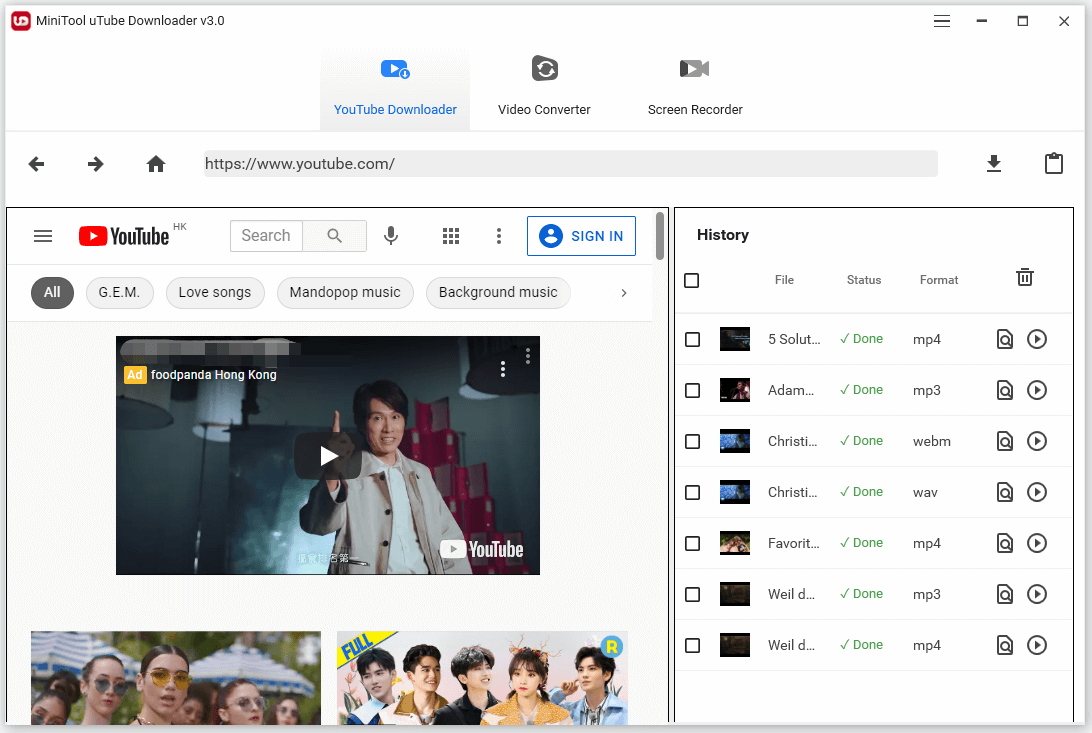The screenshot showcases the interface of the "MiniTool YouTube Downloader" version 3.0. In the top-left corner, there is a small red square logo, followed by the software's name and version. On the right side of the top bar, the interface includes the minimize, maximize, and close buttons. 

Centered on the top bar, the interface is segmented into three functional areas: "YouTube Downloader" with a YouTube icon, "Video Converter" with a file icon and a refresh symbol, and "Screen Recorder" with a camera icon. Beneath these sections, in the center of the screen, lies a search bar preset to youtube.com. To the left of the search bar are home button and navigation arrows (back and forward), while on its right side are download and clipboard icons.

The main interface is split into two large panels. The left panel, occupying most of the space, displays the YouTube homepage with the YouTube logo at the top-left corner, a central search bar, a sign-in button on the right, and several video thumbnails arranged below. The right panel, although smaller, still substantial, features a "History" section at the top-left. This section includes file status, format options, and trash can icons. Beneath these icons is a vertical list showing videos that have been uploaded to YouTube.